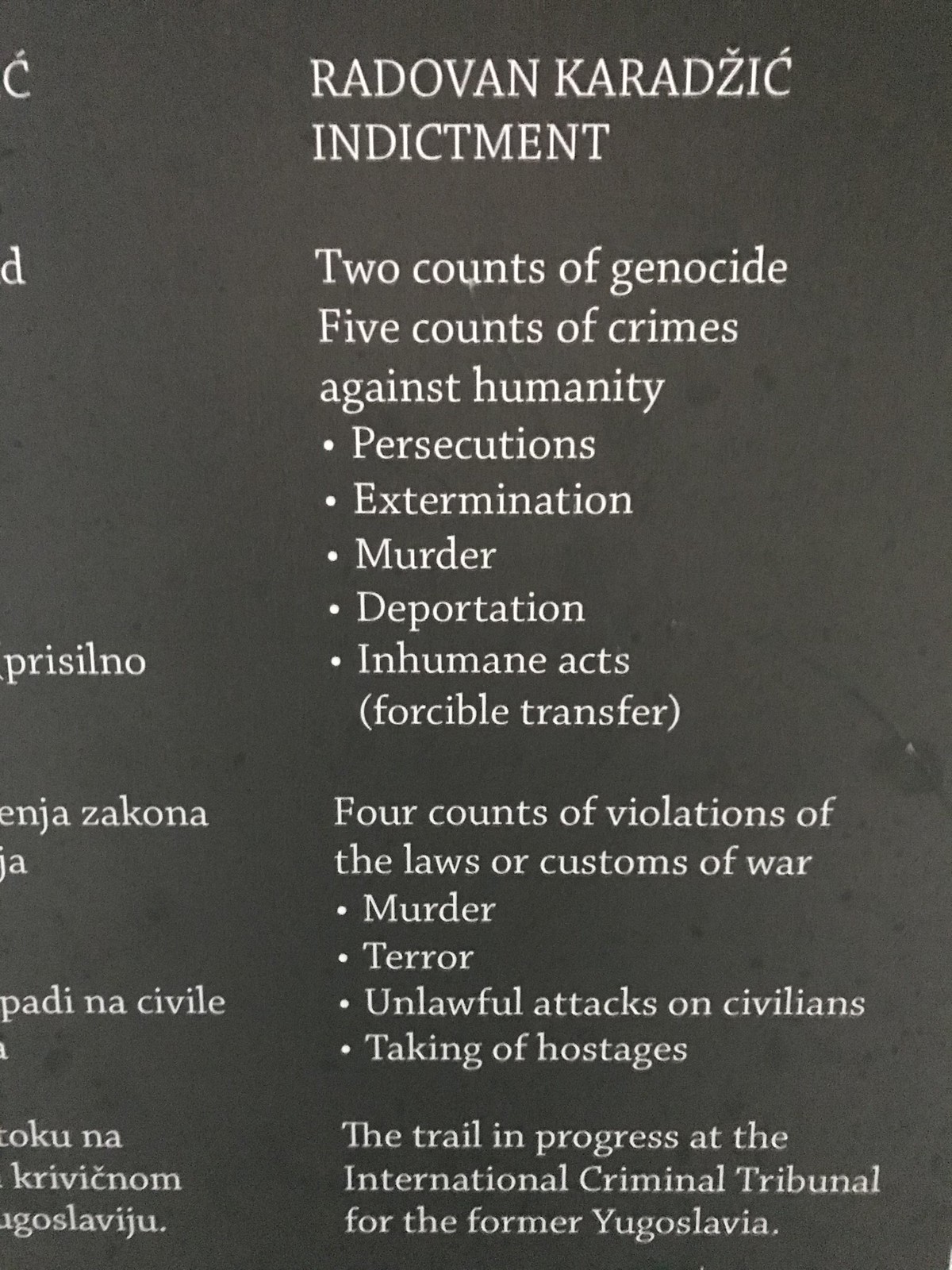The vertically aligned rectangular image features white text on a black background, primarily showcasing an indictment for Radovan Karadzic. The text is left-aligned, with a clear title at the top in all caps: "RADOVAN KARADZIC INDICTMENT." Below the title, the charges are listed: "Two counts of genocide, five counts of crimes against humanity," followed by five bullet points detailing specific charges — "persecutions, extermination, murder, deportation, and inhumane acts (forcible transfer)." Further down, the indictment specifies "four counts of violations of the laws or customs of war," with four more bullet points: "murder, terror, unlawful attacks on civilians, and taking of hostages." At the very bottom, it notes, "the trial in progress at the International Criminal Tribunal for the former Yugoslavia." The image hints at an additional column of text on the left side, partly obscured and in another language.